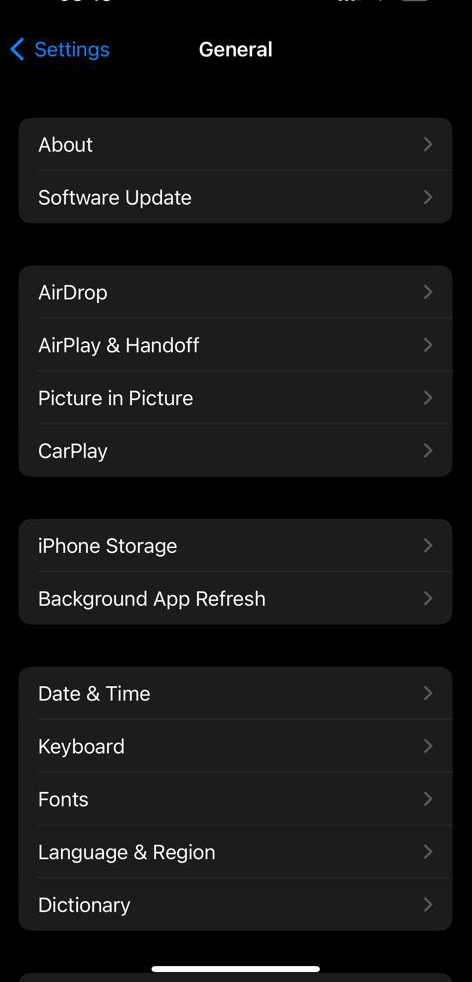The image appears to be a screenshot of a smartphone's "General" settings page. The interface features a black background with predominantly white text, making navigation elements clear and readable. 

In the upper left corner, there's a blue arrow pointing to the left beside the word "Settings," indicating a return option to the previous menu. Centrally positioned at the top is the title "General" in bold white font. 

The content is organized into sections, each demarcated by a slight variation in background shade for clarity. 

- First Section: 
  - "About" in white text, followed by an arrow pointing to the right.
  - "Software Update" in white text, also accompanied by an arrow pointing to the right.

- Second Section:
  - "AirDrop"
  - "AirPlay & Handoff"
  - "Picture in Picture"
  - "CarPlay"
  All options listed in this section are in white text with arrows pointing to the right.

- Third Section:
  - "iPhone Storage"
  - "Background App Refresh"
  Again, all items listed have arrows pointing to the right.

- Fourth Section:
  - "Date & Time"
  - "Keyboard"
  - "Fonts"
  - "Language & Region"
  - "Dictionary"
  All options are listed in white text with right-pointing arrows.

At the bottom of the screen, there is a white bar set against the dark black background, providing additional navigational context or options. 

Overall, the interface design uses contrast effectively to delineate information and options, maintaining user clarity and ease of navigation.